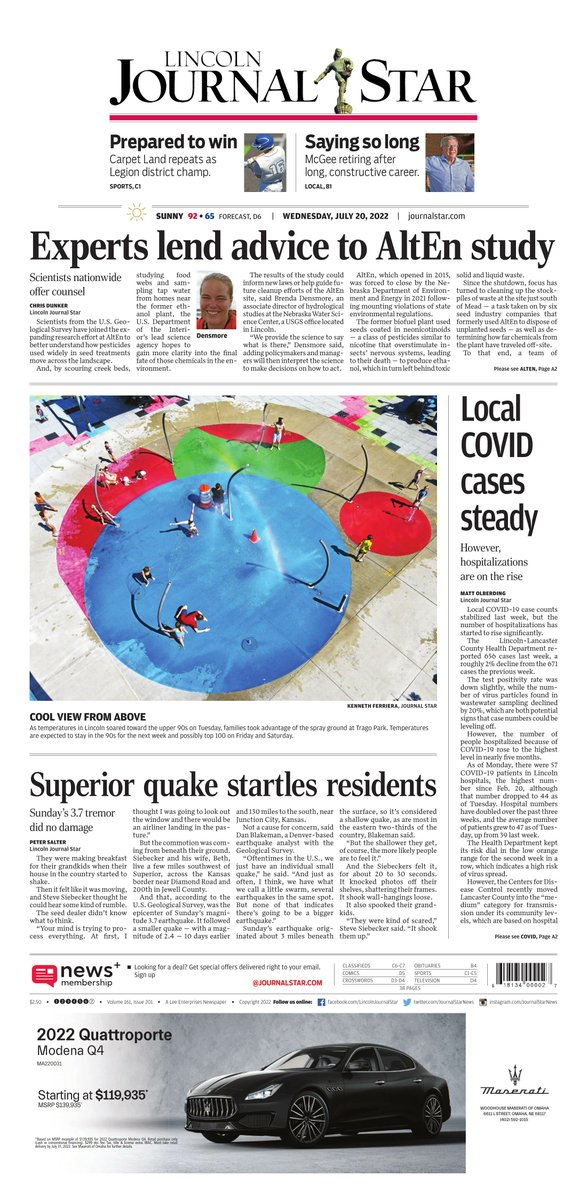The provided image is a stock photo of the Lincoln Journal Star newspaper's online front page. Dominated by a black-and-white theme, the layout features numerous rectangular text blocks, alongside intricate details of various articles. The centerpiece of the page is a vibrant, color photograph depicting an amusement park ride, captured from a bird's-eye view, featuring a dynamic array of primary colors and circular motifs.

Key headlines include:
- "Experts Lend Advice to Alt-N Study"
- "Local COVID Cases Steady"
- "Superior Quake Startles Residents"

Additionally, a prominent advertisement highlights the 2022 Maserati Quattroporte, priced at $119,935. The page also includes a piece titled "Saying So Long, McAfee," potentially referencing the passing of John McAfee, and another article titled "Prepare to Win," authored by Caprice Lance, the details of which are partly obscured.

The date indicated, April 20, 2022, situates this edition during the ongoing COVID-19 pandemic.